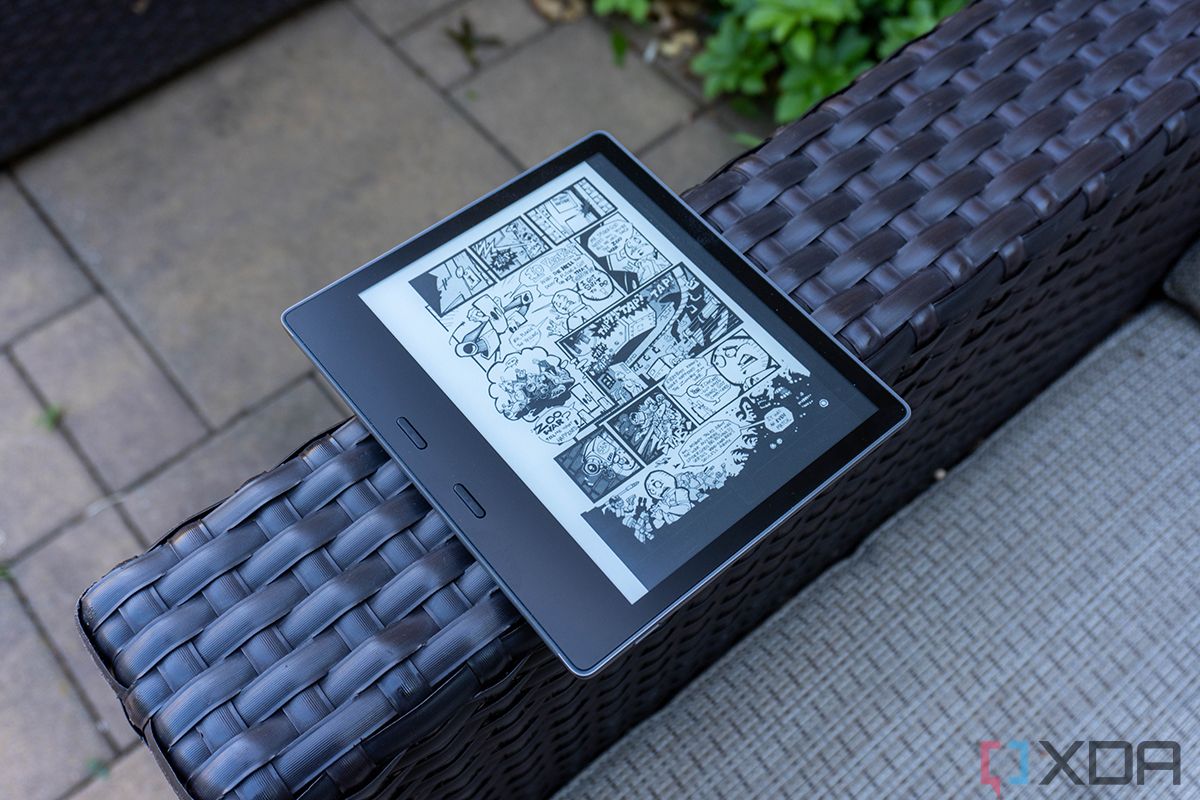The photograph, taken outdoors, features a high-quality e-reader or tablet device resembling an iPad, placed on the arm of a wicker patio lounge chair. The chair, with its black woven material and grayish-white cushion, rests on a tiled stone floor. Partially visible vegetation in the background hints at a garden or backyard setting. The e-reader's screen displays a detailed black-and-white comic strip, rich with action and dialogue bubbles. A watermark in the lower right corner features a red and blue speech bubble icon followed by the letters "XDA."